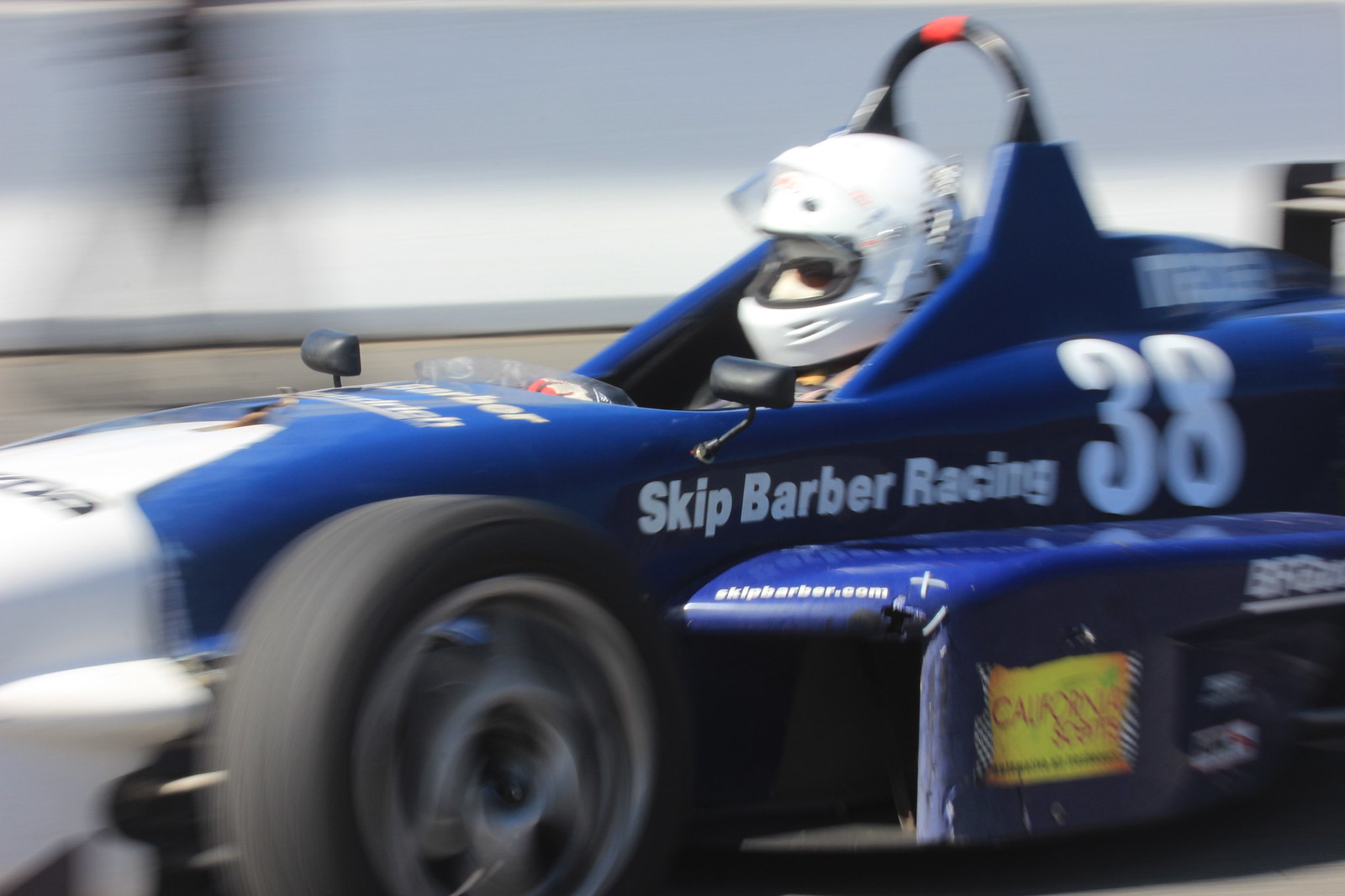The image captures a dynamic moment of an Indy race car in motion. The vibrant blue race car, which dominates the frame, features striking white accents, including a white front. Prominently displayed on the vehicle are white letters spelling out "Skip Barber Racing," right beneath the cockpit, and the large black number "38" on its side. Additional white lettering with "skipbarber.com" enhances the front view. Adding a touch of color, a yellow graphic with red text, partially blurred and reading "California something," adorns the side. The energy and speed of the scene are accentuated by the motion blur in the background. The driver, sporting a white helmet and sunglasses for eye protection, is firmly seated behind the wheel, guiding the car on what appears to be a racetrack. The image's background melds into a blurry expanse of gray, emphasizing the car's high speed and the precise moment captured mid-race.